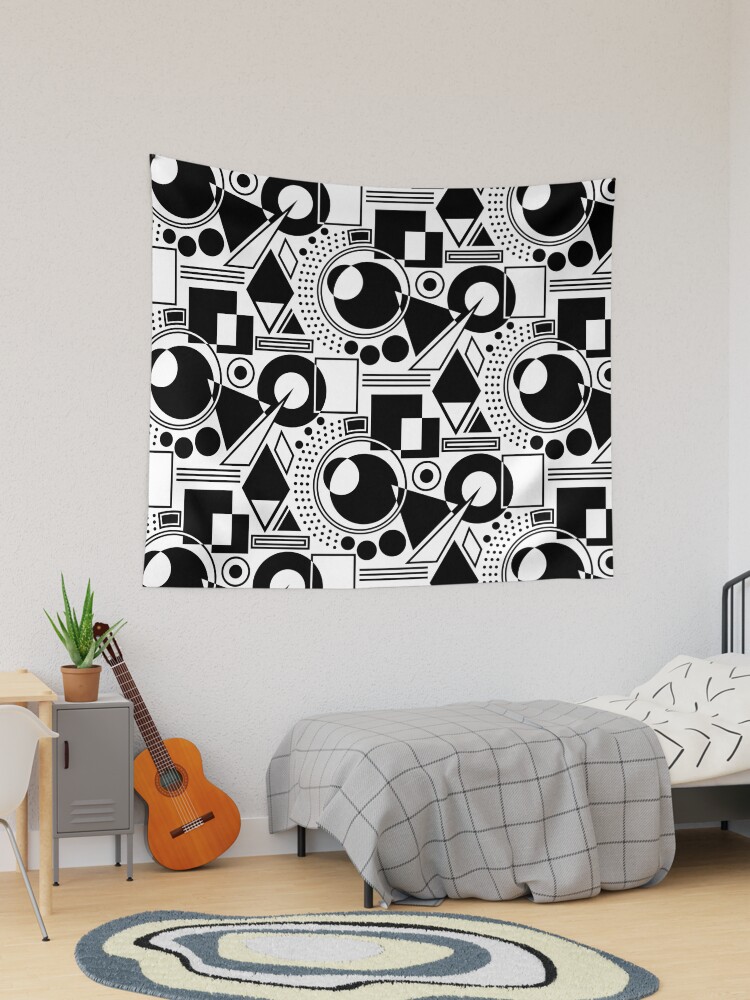The photograph captures an indoor scene, primarily focusing on a large, square-shaped tapestry mounted on a wall. The room appears to be a bedroom with solid gray walls. The tapestry, made of thin fabric, features an array of geometric shapes including rectangles, circles, and triangles in black and white against a white background. It is affixed to the wall only at the top left and top right corners. Below the tapestry, there is a twin-size bed adorned with a gray plaid comforter, white sheets, and black pillows with arrow patterns. To the left of the bed, a brown acoustic guitar leans against a small gray locker, topped with a succulent plant in a clay pot. The room also includes a circular rug placed on a hardwood floor, characterized by a series of concentric rings in gray, beige, black, and white. Additionally, a desk with a white chair is positioned to the left of the scene, contributing to the cozy, intimate ambiance of a personal living space.